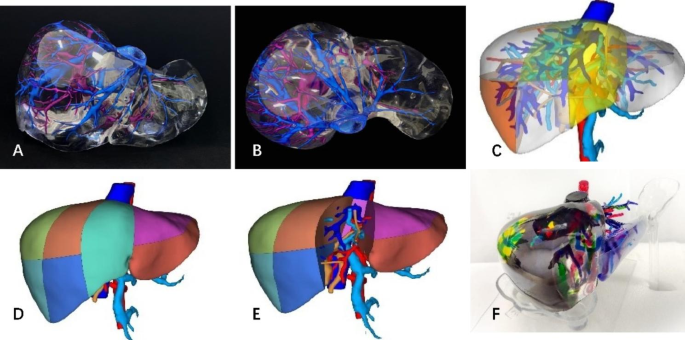The image consists of six squares, each depicting a detailed representation of the liver in various forms and perspectives. The squares are labeled A to F and are arranged with three on the top row and three on the bottom row. 

- **Square A**: Features a liver-shaped object against a black background. The organ is depicted with intricate blue and purple arteries coursing through it.
- **Square B**: Shows the same liver-shaped object from a different angle, also on a black background, maintaining the blue and purple vein-like structures.
- **Square C**: An illustration of the liver, using a vibrant palette of yellows, blues, and oranges, set against a white background.
- **Square D**: Another illustration, this time presenting the liver in a patchwork fashion of various colors including orange, blue, teal, and purple, depicting its structure more stylistically.
- **Square E**: Shows the liver cut open in the center. This illustration maintains the patchwork of colors but reveals the internal arteries, providing an inside view of the organ’s anatomy.
- **Square F**: A photographic representation where the liver appears transparent and glass-like, displaying the colored arteries within, set against a grayish background.

Through a mix of microscopic views, illustrations, and photographs, this collection showcases the liver's anatomical features in both artistic and scientific manners. The consistent use of vibrant colors and varied backgrounds highlights different aspects and perspectives of the liver's structure.